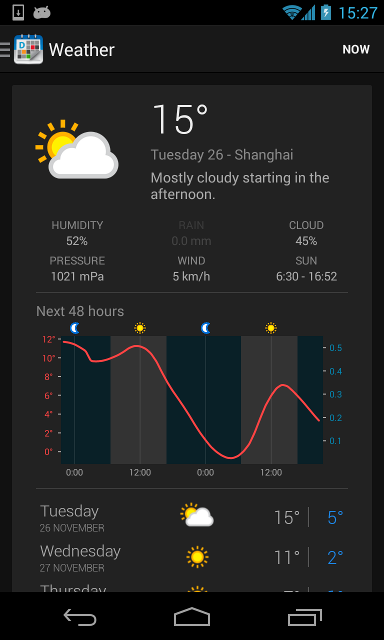**Detailed Caption:**

The screenshot, likely taken from a phone or tablet, depicts a weather app interface. In the upper left corner of the screen, there are two icons, while the upper right corner features four icons: a battery indicator, the current time displayed as "15:27," a calendar, and the weather. Below this, the app shows "NOW" indicating the current conditions.

Dominating the center of the screen, the temperature is displayed as 15°C. The date is specified as Tuesday, the 26th (month unspecified). The location is identified as Shanghai, highlighting mostly cloudy conditions expected to start in the afternoon.

Beneath this header, various weather details are organized into six categories:
- **Humidity:** 52%
- **Rain:** 0.0 mm
- **Cloud Cover:** 45%
- **Pressure:** 1021 hPa
- **Wind:** 5 km/h
- **Sunset:** 16:52

Further down, a line graph illustrates the temperature forecast for the next 48 hours. The graph starts at 12°C, dips to 0°C, and shows a rise to approximately 6°C by 12 noon the next day.

The information continues with a daily summary:
- **Tuesday, 26th November:** Daytime high of 15°C, nighttime low of 5°C (Celsius).
- **Wednesday, 27th November:** Sunny with a high of 11°C and a low of 2°C.